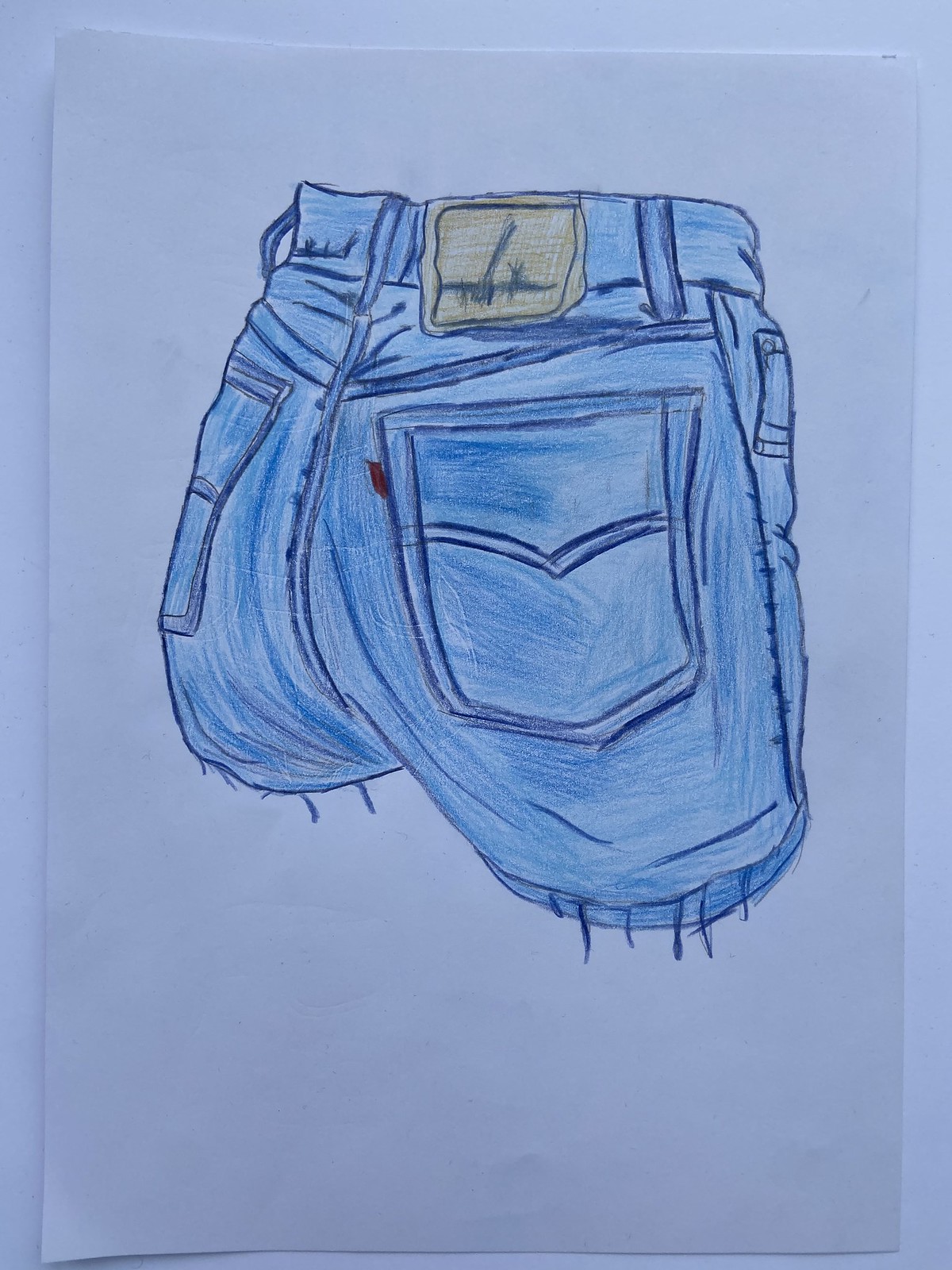This is a photograph of a detailed drawing of a pair of denim shorts, depicted from the back, on a piece of slightly dog-eared white printer paper. Both the paper and the white surface it rests on appear tinted blue due to the lighting. The sketch, created with colored pencils, features a dark navy blue outline and various shades of lighter blue to convey depth and texture. The shorts are detailed with frayed edges at the leg openings, and a brown label is positioned at the belt on the right side. The overall composition accurately showcases the distinct features of the denim shorts, including the back pockets and the characteristic fraying of cut-off jean shorts.